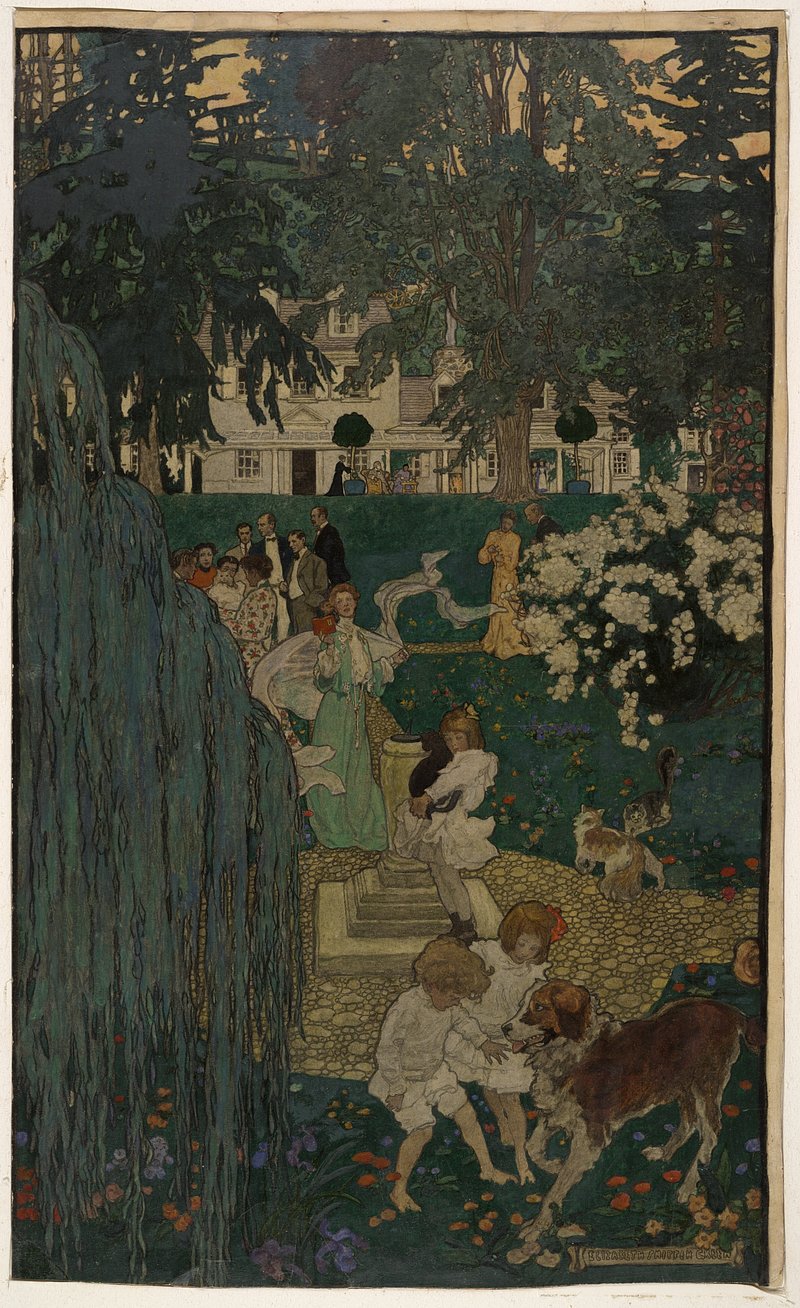This detailed painting portrays an idyllic, bustling courtyard scene outside a large Victorian-style house, framed by dark greenery that merges into a brownish-yellow sky. The white house in the background is set off by an array of trees including a bluish-green weeping willow occupying the left side. The courtyard itself is a lively scene with groups of people engaged in various activities. 

In the foreground, on the bottom right, two children dressed in white—one with long blonde hair and the other with a red bow in her brown hair—play with a brown and white dog whose tongue hangs out happily. Moving left, a girl in a white dress stands near a cylindrical fountain with a black cat in her arms, near a circular stone plaza. A small cat can be seen walking into the bushes nearby.

Central to the image is a lady in a mint green dress adorned with a flowing white veil that spans the width of the painting; she holds a red book in her right hand. Around her, a group of elegantly dressed people, women in various dresses, and men in suits and tuxedos, appear to be conversing. 

A bush with white blooming flowers stands prominently in the center right, partially hiding a couple behind it. The lush greenery, festooned with flowers of various colors, adds vibrancy to the dark tones of the artwork, illustrating a scene rich in detail and social interaction.